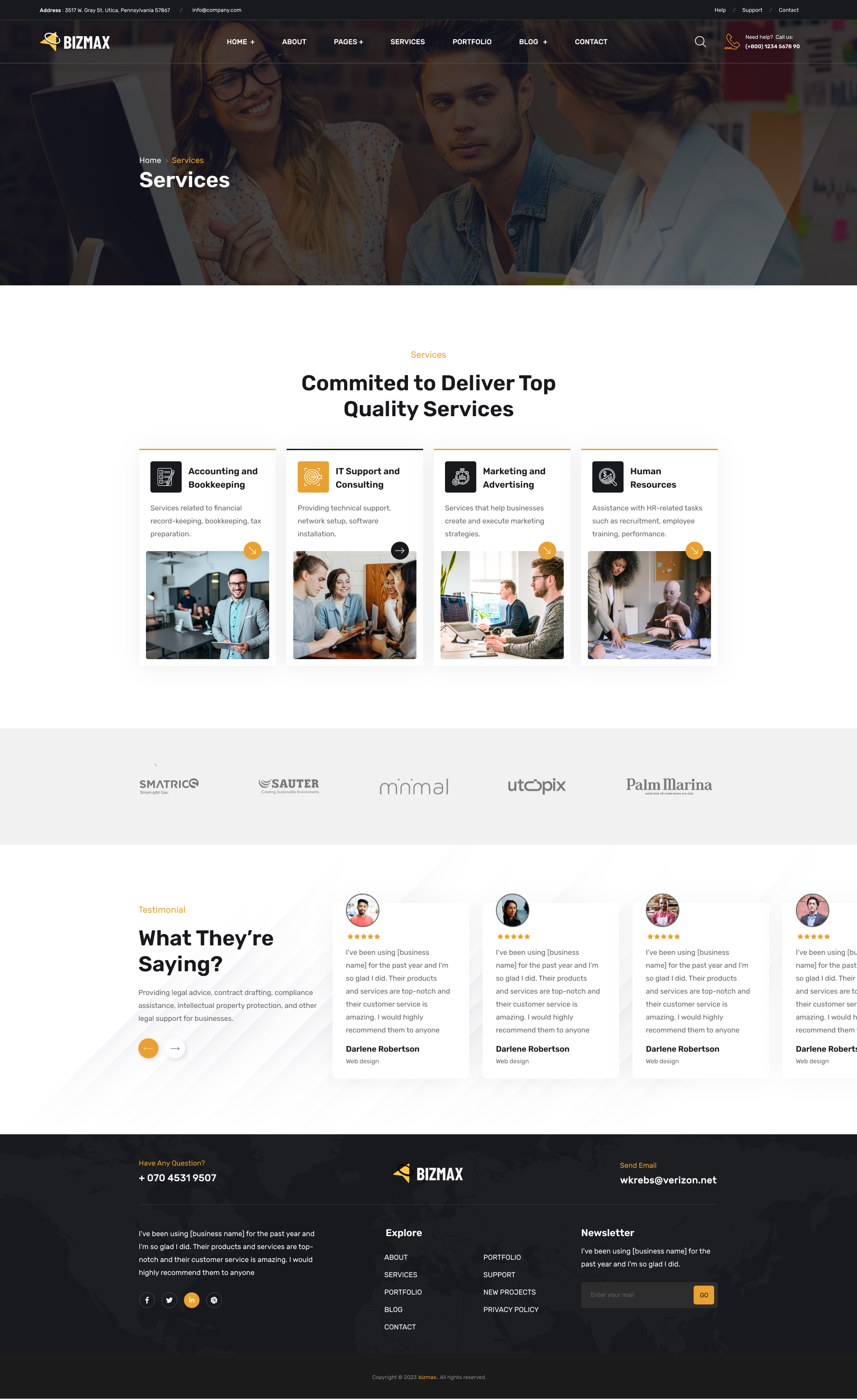This image showcases a webpage from Bismarck's website, featuring various service categories and a sleek, modern design. At the top of the page, there are navigation links including Home, Service Pages, Portfolio, Blog, and Contact. The main section displays a bold statement committing to delivering top-quality services. These services encompass several domains such as accounting and bookkeeping, financial record-keeping, tax preparation, IT support and consulting, which includes technical and network support and software installation. Additionally, marketing and advertising services are offered to help businesses develop and implement effective marketing strategies. Furthermore, the company provides human resources assistance, covering tasks like recruitment, employee training, and performance management. At the bottom of the page, sponsors like Smartrick, Salter, Minimal, Utopix, and Palm Arena are prominently displayed. The color scheme of the page features a combination of orange, black, and white, lending it a clean and professional appearance.